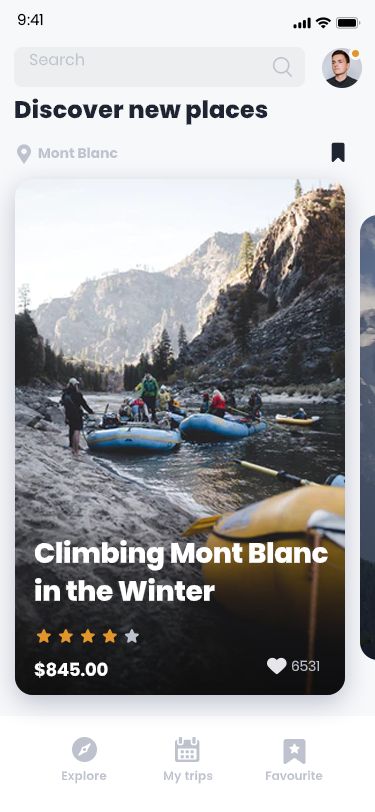The image depicts a screenshot from an iPhone. In the top right corner, three icons are visible: the signal bar, Wi-Fi symbol, and battery icon, the latter showing the battery level with a black fill but without a numerical percentage. The current time displayed is 9:41.

Below these icons, a gray search box is situated centrally, featuring a magnifying glass icon on its right side. Adjacent to the search box on the right is a profile picture of a man with black hair, slightly turned to the left, with a small orange circle above his head.

Beneath the search box is a text that reads "Discover new places" followed by "Mont Blanc," the text being in a gray color. Dominating the majority of the screen below this text is an image showcasing a picturesque scene of people in boats amidst mountains.